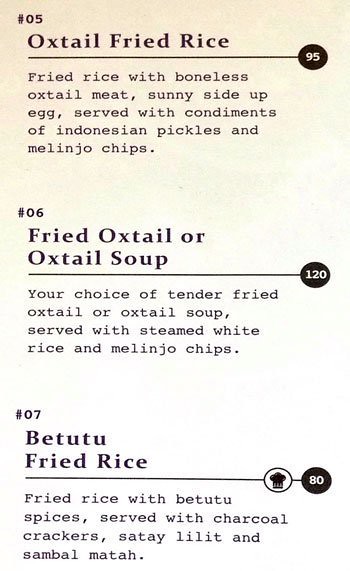The image showcases a light pink cardstock menu featuring three items, numbered 5, 6, and 7. Item number 5 is Oxtail Fried Rice, described as fried rice with boneless oxtail meat, accompanied by a sunny-side-up egg, and served with Indonesian pickles and chips, priced at 95. Item number 6 offers a choice between Fried Oxtail or Oxtail Soup, both served with steamed white rice and chips, priced at 120. Lastly, item number 7 is Betutu Fried Rice, which is fried rice with betutu spices, served with charcoal crackers, satay lilit, and sambal matah, priced at 80. A small symbol resembling a muffin is next to the description of this item. The text appears to be in black, printed on what seems to be an older or slightly dated menu.